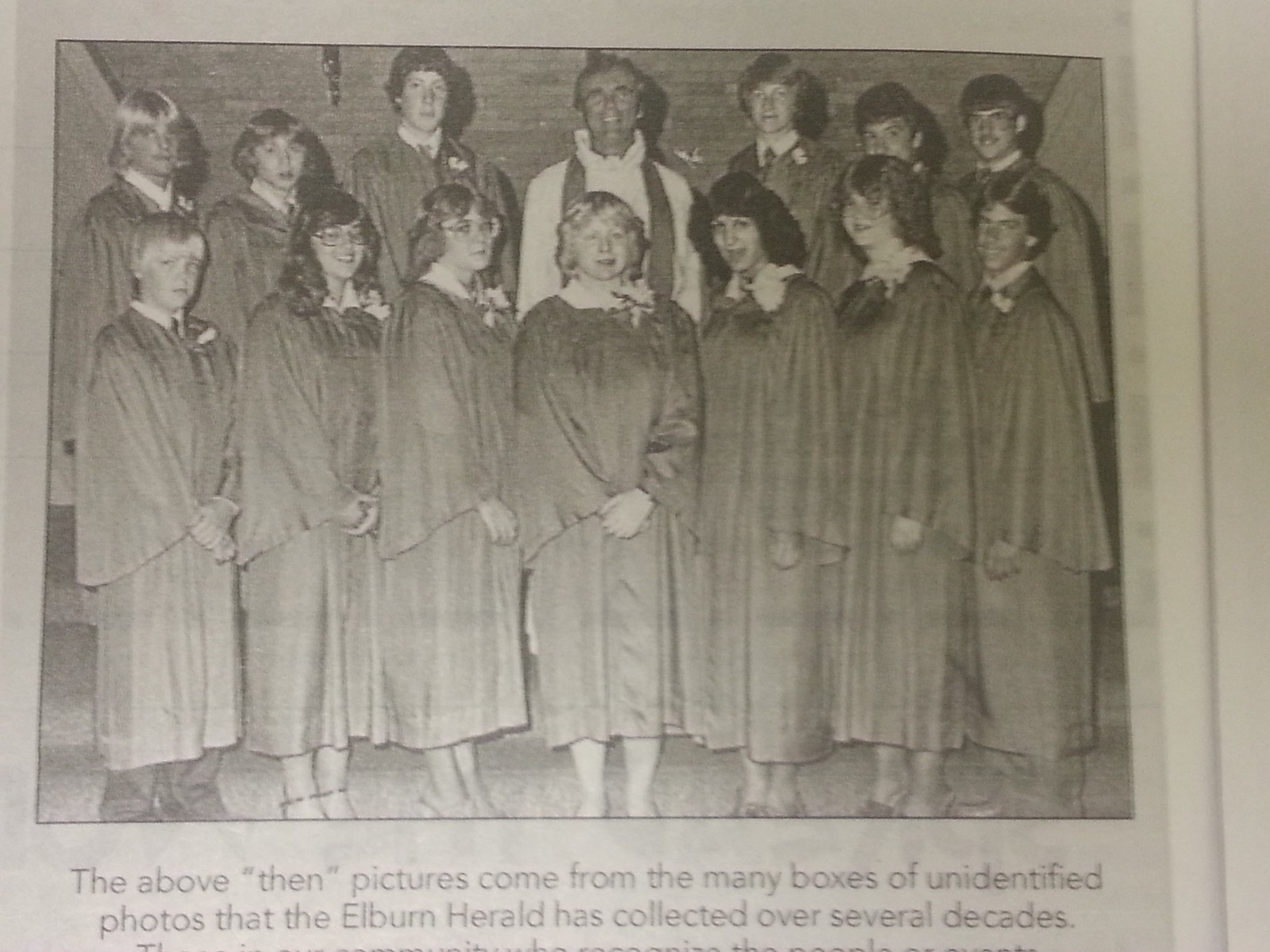This black and white image, most likely from the 1960s or 70s, captures a group of 14 individuals standing in two rows. The group consists of boys and girls, all clad in what appear to be graduation robes. The boys are wearing shirts and ties underneath, while the girls have white collars; each person is adorned with a flower. Their hair is carefully styled for the occasion. Smiling towards the camera, the only adult figure, positioned centrally in the back row, stands out with a distinct attire—a white robe featuring a darker sash. This photograph, showing an older man and 13 younger individuals, forms part of the many unidentified images that the Elburn Herald has amassed over several decades, as indicated by the partially visible text below the image.